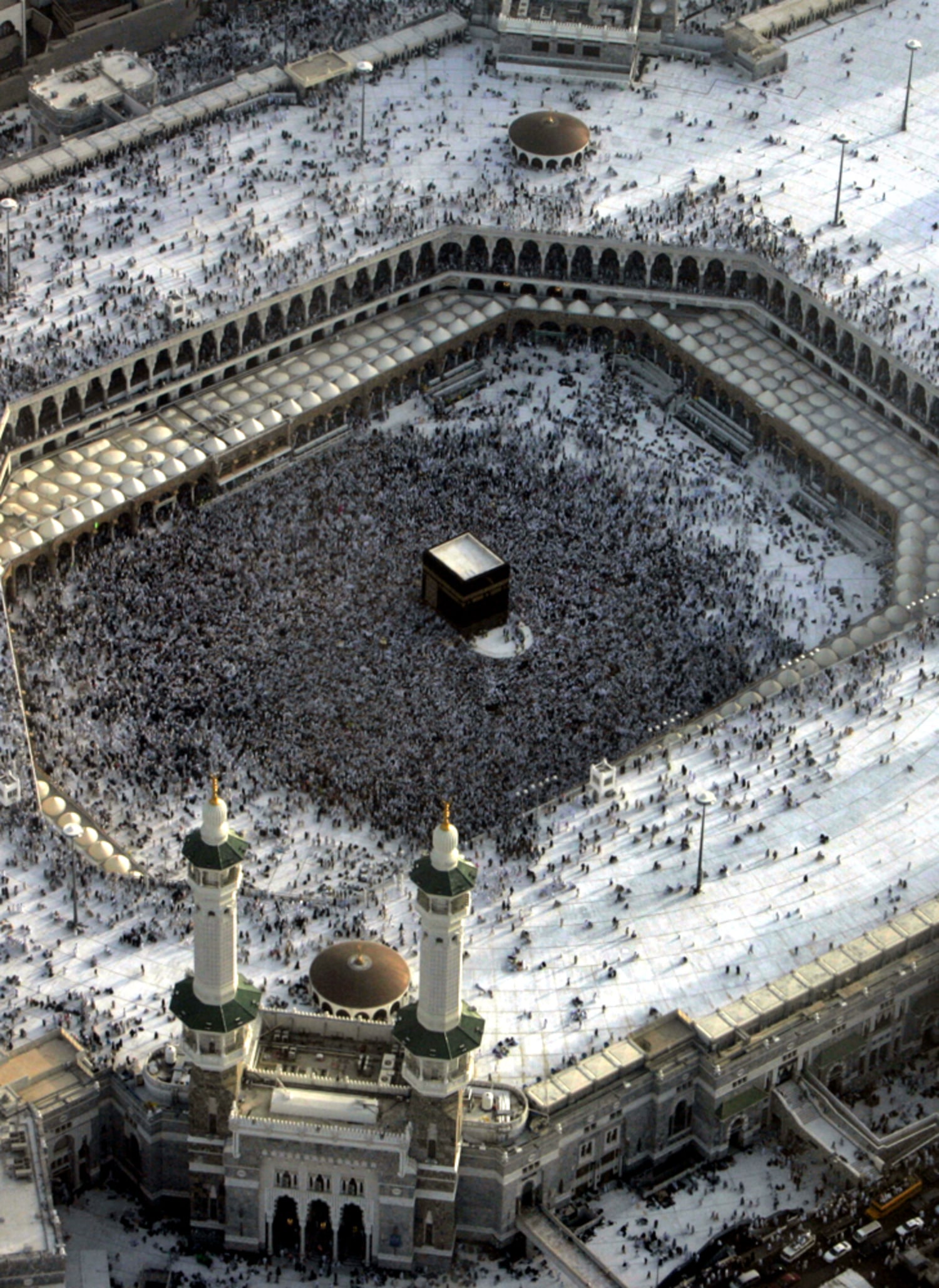Captured from a high-altitude aerial perspective, this photograph presents a breathtaking view of a grand structure, likely a mosque, but eliciting elements reminiscent of a castle or cathedral. Dominating the scene are two towering spires adorned in white and green hues with glistening gold tops, giving the facade a somewhat Gothic feel. Below, the vast courtyard, possibly associated with the Hajj pilgrimage, is densely packed with people who appear like tiny ants from this height, emphasizing the immense scale. The central focus within the courtyard is a large square building, believed to be the Kaaba, surrounded by an immense crowd. This crowd spills into the outer areas, revealing a strategically arranged pathway bordered by what appear to be tent-like structures. The structure’s exterior includes prominent features like three arched doorways and towering columns, each topped with what resembles lighthouses. The building's periphery showcases additional smaller entrances, equipped with ramps and stairs, indicating access points. The stone architecture is crisply outlined against snow-covered surroundings, and the fringes of the image show a glimpse of the street below, dotted with cars, adding to the understanding of the photo’s vast scope and detailed intricacies.